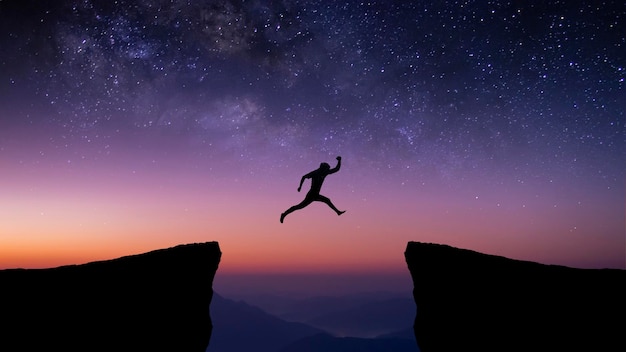A 3D rendering depicts a dramatic scene of a silhouetted figure jumping a short distance between two sheer, black cliff sides that emerge from the bottom left and bottom right corners of the rectangular image. The figure occupies the center of the image, frozen mid-air with one arm extended behind and the other raised, legs spread in a dynamic leaping pose. The background reveals a captivating night sky, transitioning from a dark purple overhead, dotted with white stars and planets, to a lighter orange hue as it meets the horizon. Multiple purple-hued hills can be discerned in the distance, contributing to the image's sense of depth and the low light ambiance.